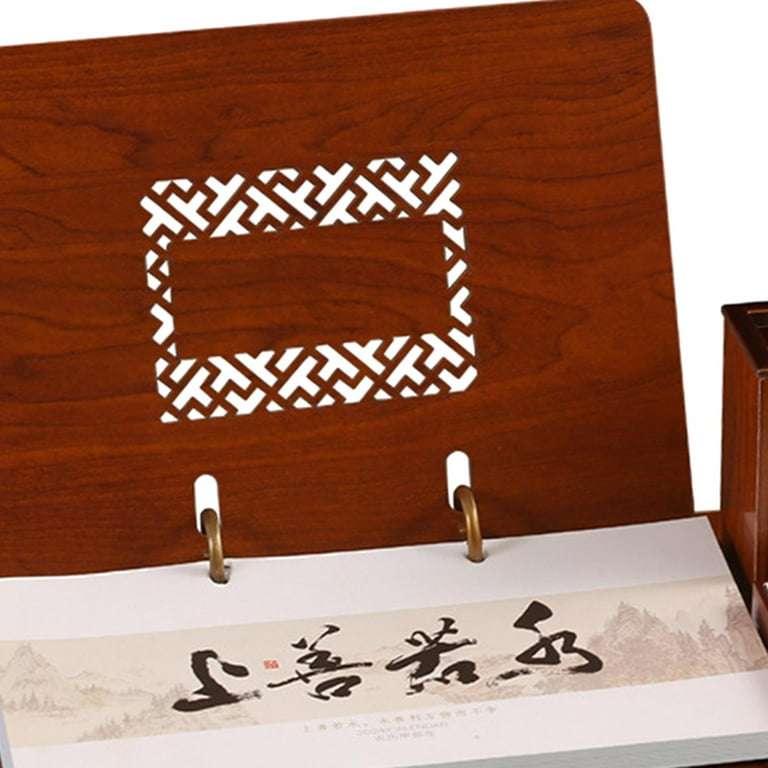The image features a vertically rectangular photograph, taken indoors with artificial lighting, giving it a staged and artistic appearance. Central to the image is a binder with gold rings, holding yellowish paper. The cover of the binder is crafted from dark, well-polished wood, occupying the upper two-thirds of the photograph. The wooden cover is intricately designed with a geometric, Tetris-like pattern of interconnecting white capital T's framing a solid rectangular wooden center. The bound pages appear to be a long rectangular piece of paper, with white borders on the top and bottom. The central section of the paper displays an image of mountains and architecture, overlaid by black calligraphy consisting of four blocks of characters, with additional, smaller text below. The overall setup resembles a sophisticated paper storage device, possibly intended for preserving important calligraphy or photographs.